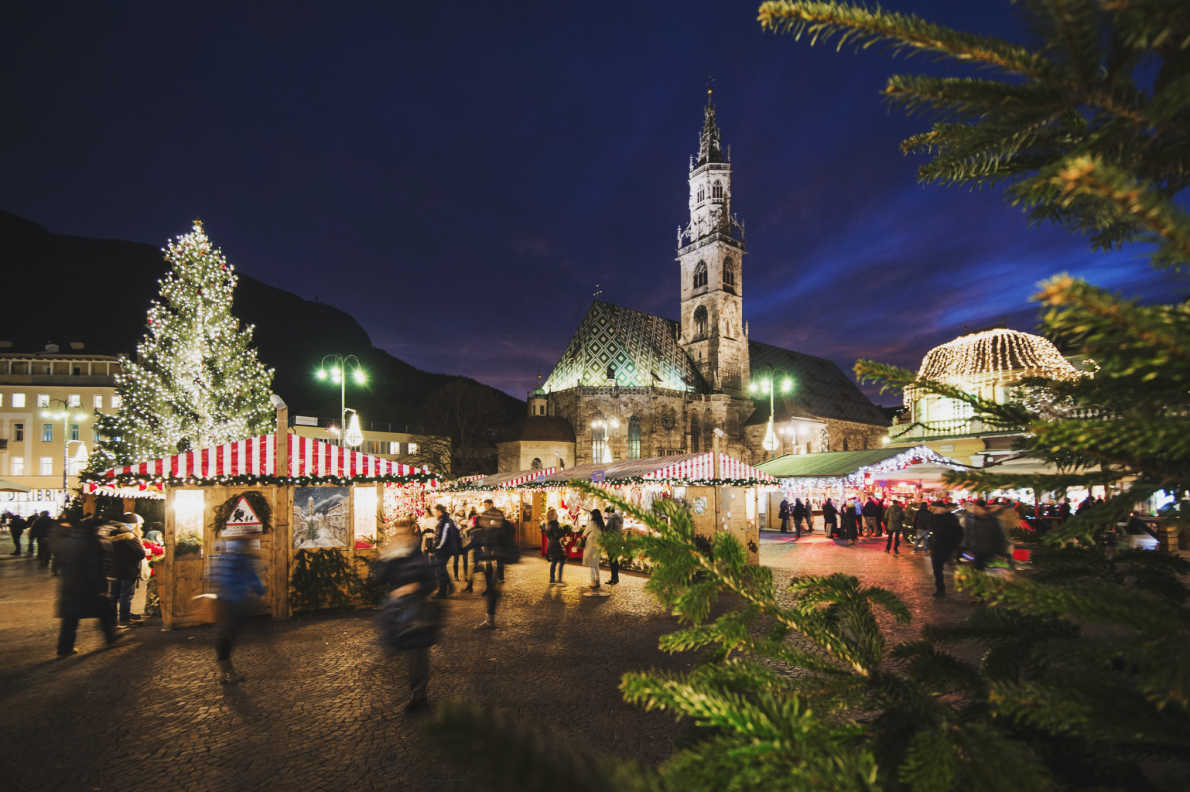The image captures a bustling Christmas festival set in the picturesque town square of what appears to be a European village, likely in Scandinavia or Germany. Dominating the background is a historic cathedral with a geometric patterned roof, standing majestically against a dark blue twilight sky, tinged with streaks of lighter blue where the sun has recently set. In the foreground, a beautifully decorated Christmas tree adorned with white lights and possibly red ornaments stands on the left, while the edges of a lush pine tree, slightly out of focus, occupy the right side.

Numerous wooden booths with festive red and white candy cane-striped roofs line the square, teeming with vendors and attendees. One stand in the distance is notable for its green corrugated metal roof. The buildings in the background are similarly adorned with strings of white Christmas lights, adding to the enchanting atmosphere. The street lights give off a greenish hue, further casting a magical glow over the lively scene. The crowds, though blurred, convey a sense of constant movement and excitement, as people mill around, enjoying the holiday festivities in this cozy, European-style village setting.